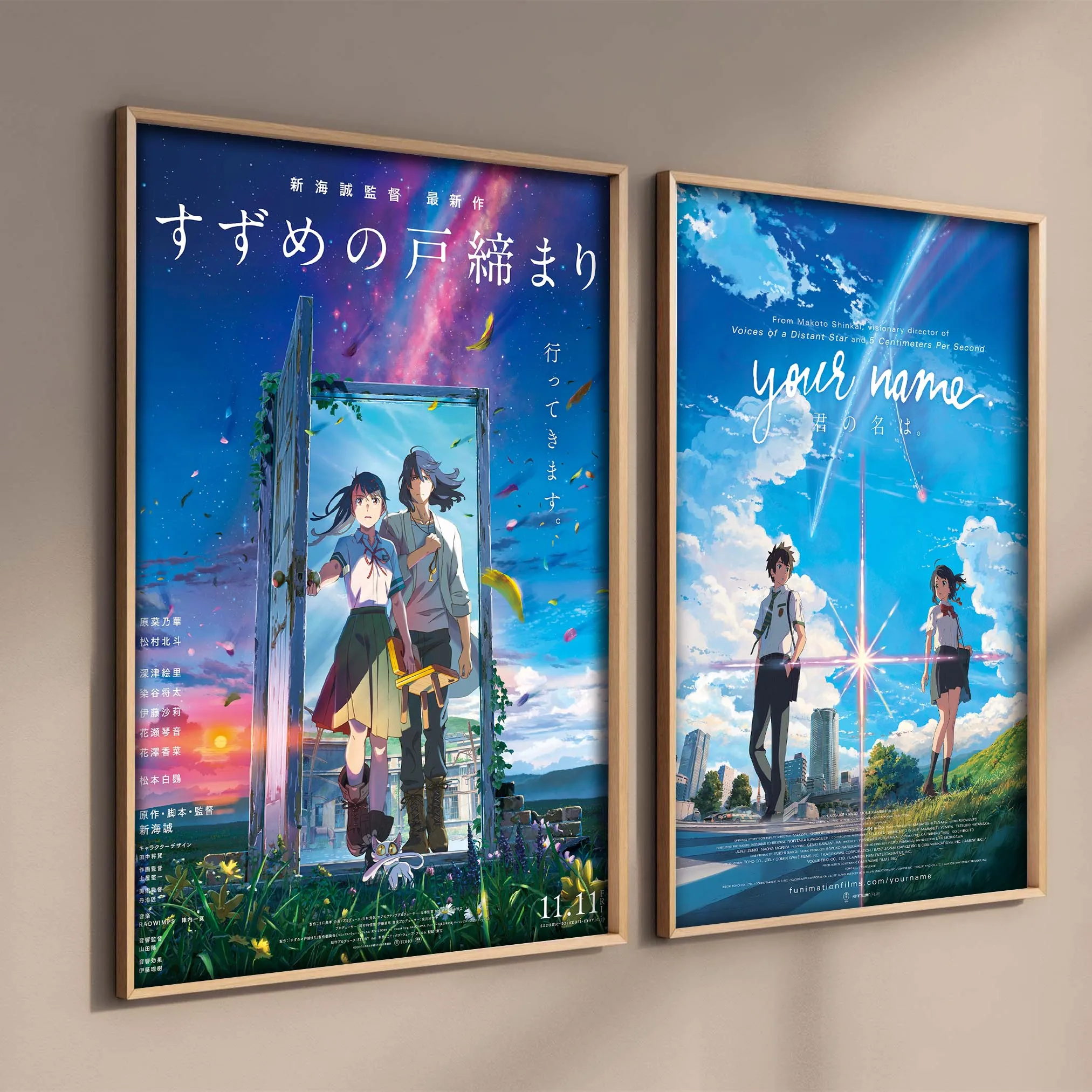In this image, two framed anime posters are mounted side by side on a beige or tan wall. The posters appear to advertise the Japanese film "Your Name." Both posters display vibrant artwork featuring the film's main characters but present different scenes. 

In the first poster, a young woman with short black hair, dressed in a white school uniform with blue-green stripes and a green skirt, opens a door revealing a blooming garden with yellow flowers and lush green grass. Behind her, a young man with short black hair, wearing a green vest, white undershirt, green pants, and brown boots, follows her. The sky in the background is dramatic with streaks of purple, blue, pink, and red, indicating a sunset with an orange sun. Japanese text, likely the title and credits, is displayed prominently.

The second poster shifts to a cityscape setting. Here, the characters wear different school uniforms: the girl has her hair in a ponytail, wearing a white top with a red tie, a black skirt, and brown shoes; the boy is seen standing on a crosswalk with skyscrapers in the background. The sky is bright cyan with some clouds and a prominent star. The English title, "Your Name," is visible at the top, along with credits to Makoto Shinkai, the director known for "Voices of a Distant Star" and "5 Centimeters Per Second." Both posters encapsulate the film's thematic contrasts between rural and urban settings.